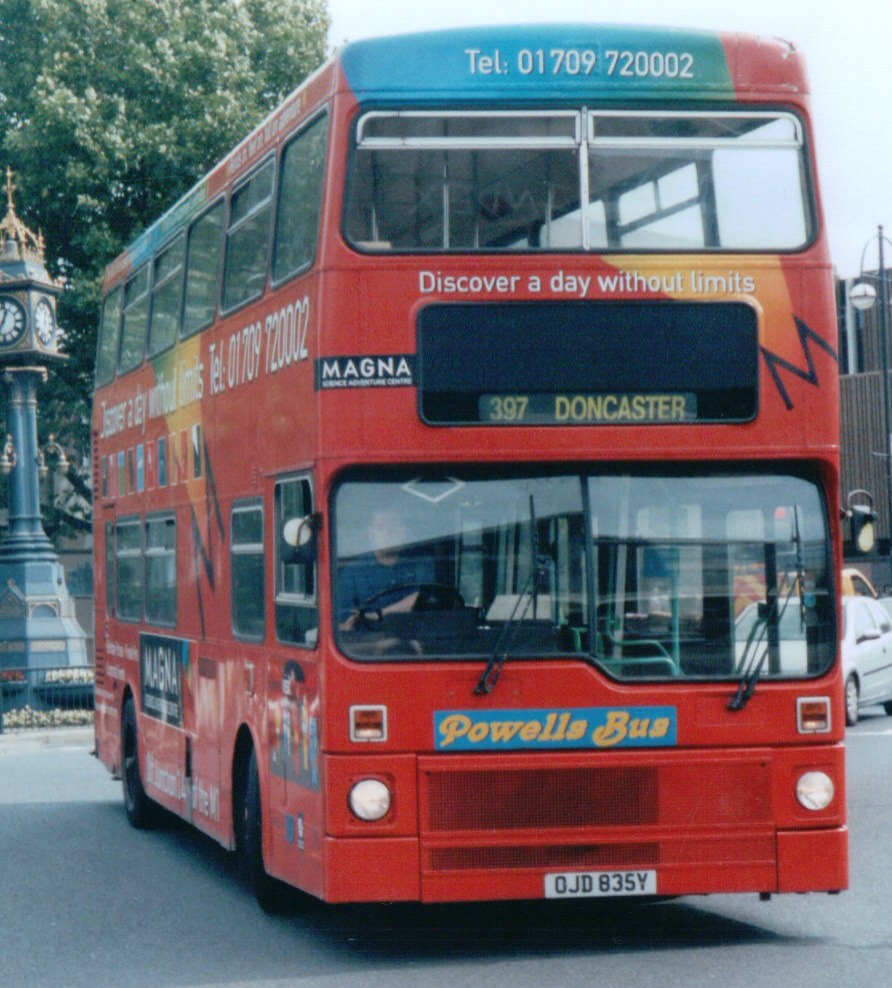In the image, a vivid red double-decker bus dominates the frame, proudly bearing the number 397 with its destination labeled as Doncaster. The bus features distinct blue trim and a mix of white lettering for various advertisements. The top front panel reads, "Discover a Day Without Limits," and below that, just above the large windshield wipers, it displays the bus's number and destination. Below the driver's window, in a blue box with yellow font, it reads "Powell's Bus." The male driver, dressed in a blue shirt with short dark hair, is visible through the windshield, and the bus carries a white license plate marked OJD 835 Y. To the left of the bus, a picturesque clock tower, painted light blue and surrounded by lush leafy trees, adds charm to the scene. On the right side, a glimpse of the street reveals a small passenger car and the edge of a brown building. The bus, with its prominent red and blue color scheme, stands out against the light blue sky, contributing to a lively urban atmosphere.